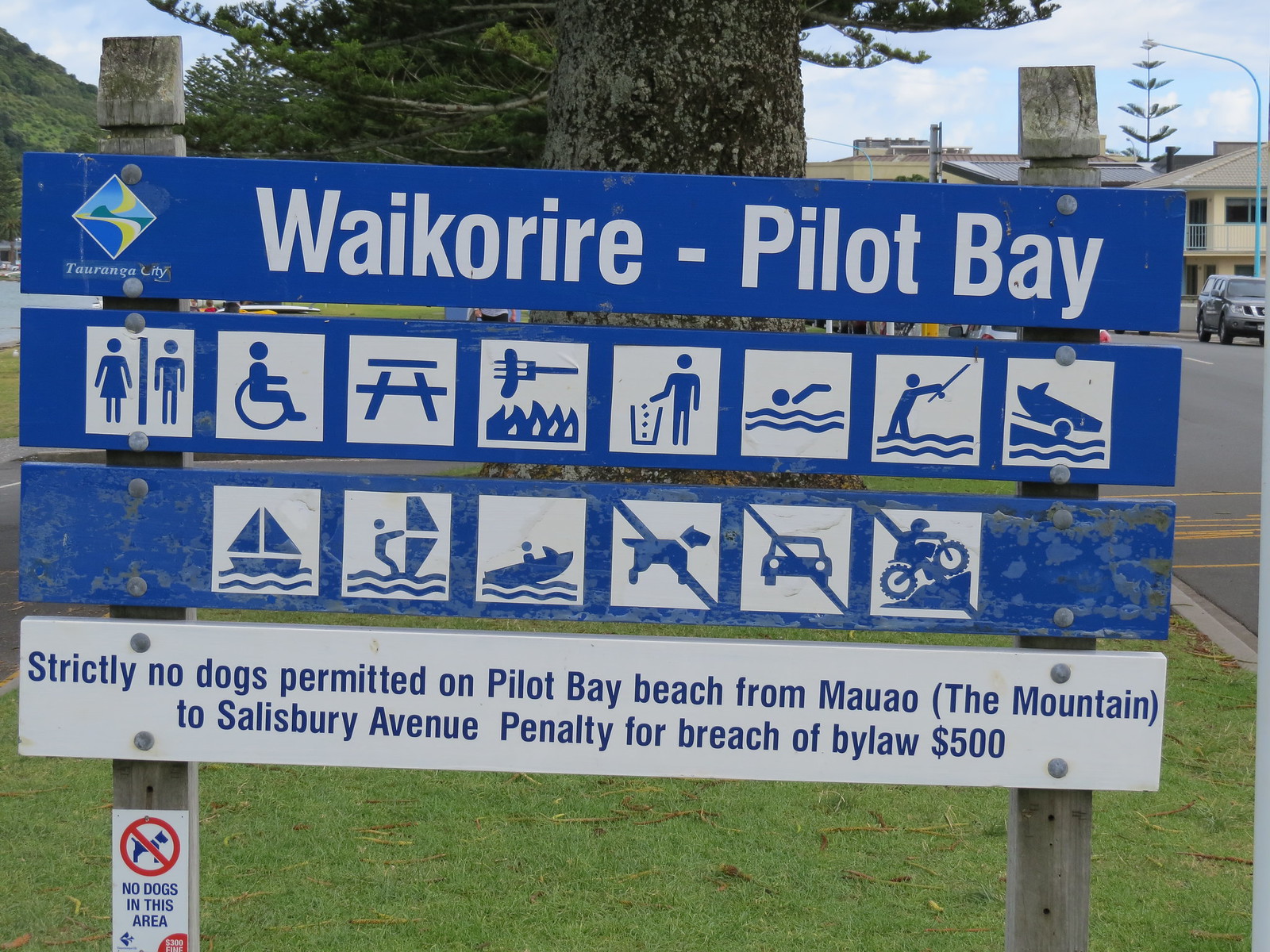Centered in a grassy area, this horizontally aligned rectangular image showcases a blue and white sign marking Waikoree - Pilot Bay. It stands prominently on two vertical wooden posts, within a small grass island between two two-lane streets. In the background, to the upper left, is a hill densely covered in trees, with a large tree trunk and green branches more prominently visible in the mid-ground. To the right, part of a street featuring a gray SUV, a light pole, and a distant two-story structure, possibly a house or business building, can be observed.

The sign itself is detailed with multiple elements:
- At the top, it reads "Waikoree W-A-I-K-O-R-I-R-E - Pilot Bay," with a diamond-shaped logo depicting a yellow and white road curving around a hill.
- There are two rows of square images illustrating various symbols, such as male and female figures, a wheelchair, a picnic table, a barbecue with utensils, a person throwing away trash, and swimming.
- A white board at the bottom states, "Strictly no dogs permitted on Pilot Bay Beach from the mountain to Salisbury Avenue. Penalty for breach of bylaw $500."

Additionally, affixed to the left wooden post, another sign clearly indicates, "No dogs in this area," featuring an outlined dog encircled with a red slash.

The vibrant colors captured in the image include shades of green from the grass and trees, blue from the sign, white and tan text, and red detailing on the dog prohibition sign, all set against a bright, daylight outdoor scene.